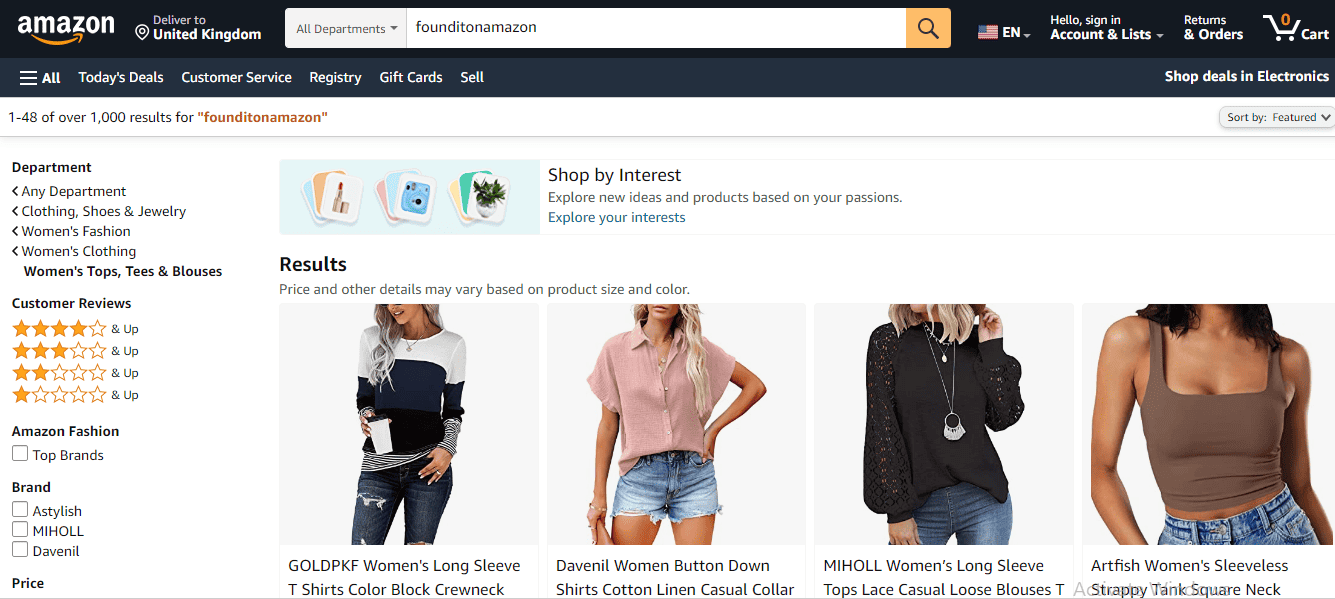The image depicts the Amazon UK homepage, showcasing various elements and navigation options. The upper section features a long, black rectangle, which includes the Amazon brand name situated in the left upper corner. There is a search bar on the left side that displays the text "All Departments" and has a small yellow square with a magnifying glass icon for search functionality. To the right of the search bar, there is an American flag icon accompanied by the uppercase text "EN," indicating the language setting.

Adjacent to these elements, the interface greets the user with "Hello, Sign In," alongside a notification that the cart has zero items. The page also displays a search result summary, stating "1-48 of over 1,000 results found on Amazon."

Below this summary, the search results begin with images of various women modeling different clothing items. The first image presents a woman wearing a blue and white long-sleeve shirt, paired with distressed jeans, and holding a coffee cup. The next image features a woman dressed in a cotton-linen pink button-up shirt and jean shorts. Following this, another woman with short blonde hair is shown wearing a long-sleeve black shirt adorned with lace sleeves; the caption beneath reads "Tops Lace Casual Loose Blouses." The final image displays a woman in a cropped brown tank top with the caption "Strappy Tank Square Neck" underneath.